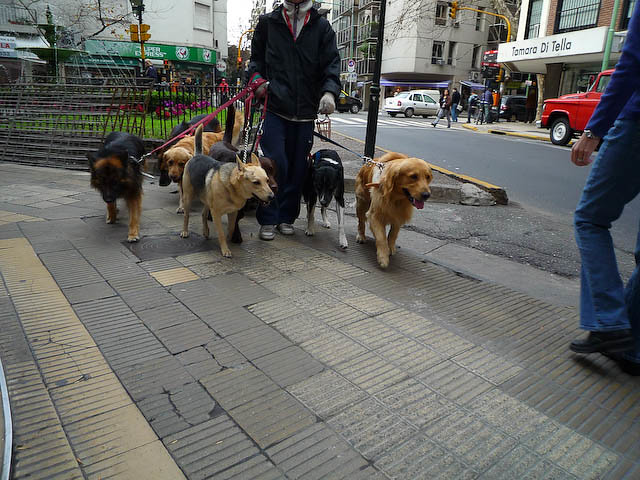In the photograph, a dog walker, dressed in a combination of a heavy black coat, either blue or brown pants, sneakers, and a possible sweatshirt overlayed with a jacket, navigates a bustling city street. Seven or eight dogs, a mix that includes Golden Retrievers, possibly some Labradors, a black dog with distinctive white paws, a dark black dog, and two that might be Australian Shepherds or Malamutes, are attached to red and brown leashes held in his right hand. His right hand is mittened, while his left seems to grip a wired object. The scene is set against a cobblestone sidewalk, and a man in jeans and a blue jacket with a watch is walking towards the dog walker, mostly out of frame.

Across the street, there's a red truck parked near a building with a sign that reads "Tommaro Di Tello," suggesting an Italian locale. Near the dog walker, a small gated park area with green grass and flowers contrasts with the bare trees, hinting at the winter season. The street brims with activity, as people cross a nearby busy intersection marked by traffic lights, and a white car navigates through. Despite being a detailed snapshot of urban life, the photo cuts off part of the central figure, providing a candid, dynamic glimpse into the cityscape.